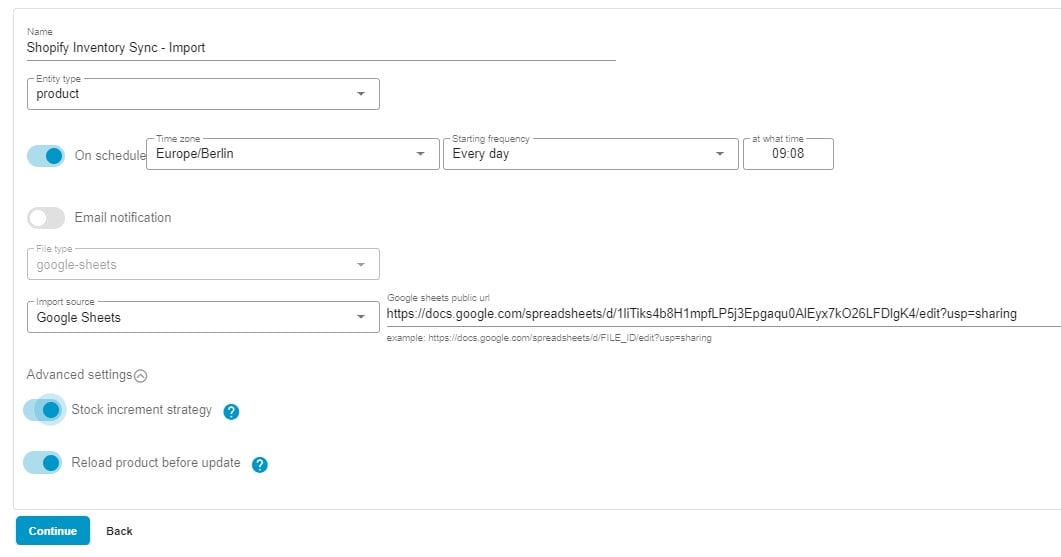**Detailed Caption:**

The image showcases a user interface designed for importing product data into Shopify using a PHP-based app named "Majora's Sink". The import settings are configured to pull the entire product catalog from a specified Google Sheets document. The frequency of this import is set to occur daily at 09:08 AM. 

Key elements within the interface include options to toggle email notifications and specify the file type as Google Sheets. The import source is confirmed to be a Google Sheets document, with the text "Google Sheets" displayed in black font.

The provided public URL for the Google Sheets document is: 
"https://docs.google.com/spreadsheet/g1litakes4bh1mpflp5j3eppgaqu2aieyix7k026ltlgk4/edit?qsp=sharing". 

Additionally, there is an example URL displayed: 
"https://docs.google.com/spreadsheet/g/https://docs.google.com/d/h/file_id/edit?qsp=sharing". 

Advanced settings allow the user to toggle options such as "reload product before update". At the bottom left of the interface, there are two blue buttons labeled "Continue" at the center and "Back". The configuration is specifically catered to Shopify platform users.

This detailed interface allows for meticulous management and automation of product data imports, enhancing efficiency for online store owners.